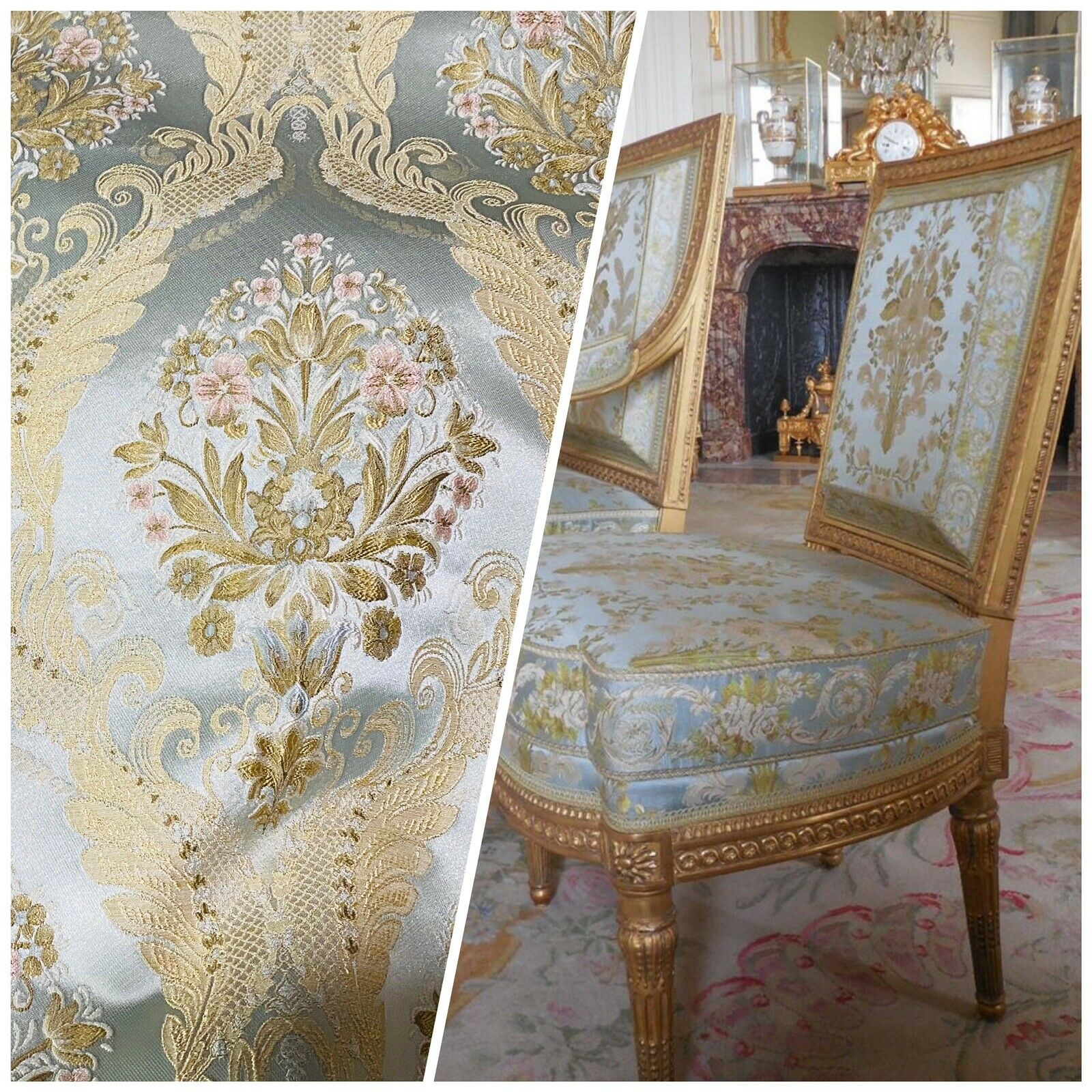This image is a split-screen composition divided diagonally from top right to bottom left. On the left side, there is a close-up view of the intricate embroidery on an antique, royal-looking chair. The fabric features a light blue or silvery background adorned with highly detailed floral and scrollwork designs in gold, pink, and white. The embroidery is accentuated by a silver background, showcasing an intricate damask pattern with ivory lacework.

The right side of the split screen reveals a broader view of an antique living room space. The main focus is a cushioned chair without armrests, boasting a golden wooden base and legs. This luxurious chair, with its rectangular back and richly-tooled wooden frame, is accompanied by another chair with armrests in the background. Both chairs rest on a floral-patterned carpet. Behind them stands an elegant marble fireplace with gold accents, adorned with a mantel clock, crystal chandelier, and vases encased in protective display cases. A large mirror hangs above the fireplace, reflecting more of the room's opulent decor.